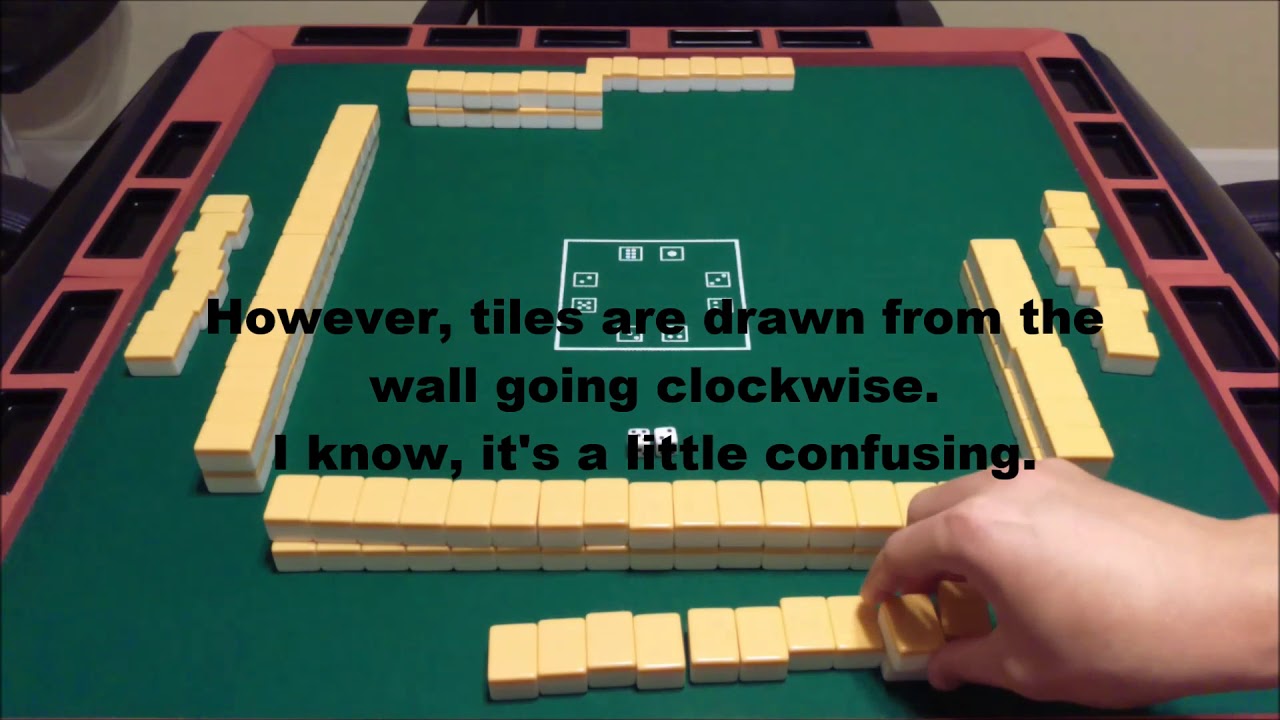The photograph captures a game board set up for a tile-based game on a green felt square table with a red border and additional black detailing along the edges. The tiles, resembling small off-white to yellowy-hued cubes, are arranged to form four walls in a square shape. Behind this square formation, extra tiles are lined up. The center of the table features a white square marked with different dice values, showcasing numbers one through six, indicating different dice rules. A pair of dice is also seen on the table. Overlaid in black text in the middle of the image, it reads, "However, tiles are drawn from the wall going clockwise. I know, it's a little confusing." Additionally, a hand is visible from the bottom right corner, holding several tiles, suggesting an ongoing move in the game. The overall appearance suggests it might be an instructional screenshot or a setup for demo purposes, emphasizing both the tile arrangement and the dice rules central to gameplay.